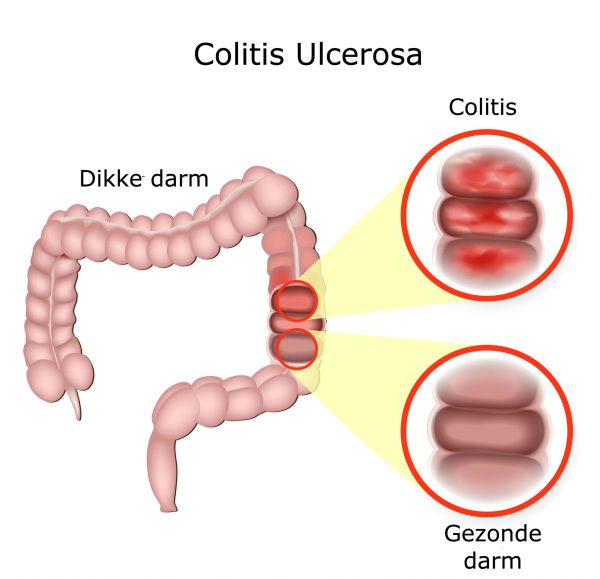The image is a scientifically-styled, graphical depiction of intestines, likely from a medical textbook or journal, illustrating colitis ulcerosa. Prominently, at the top center in black text, it states "Colitis Mucilorosa." Below this, two outlined circles filled with red and yellow tones highlight inflamed areas of the intestine, showing the severe redness indicating colitis. These circles zoom into sections of the pink, tubular intestine, labeled "Dikkedarm" at the top. The more inflamed section is denoted as "Colitis" in one bubble, while the relatively healthier segment is annotated as "Gizonde Darm." The diagram is educational, using colors such as white, pink, red, and yellow to differentiate between normal and inflamed tissues, with "Dikkedarm" situating itself prominently above the intestine, marking it as a significant anatomical term.